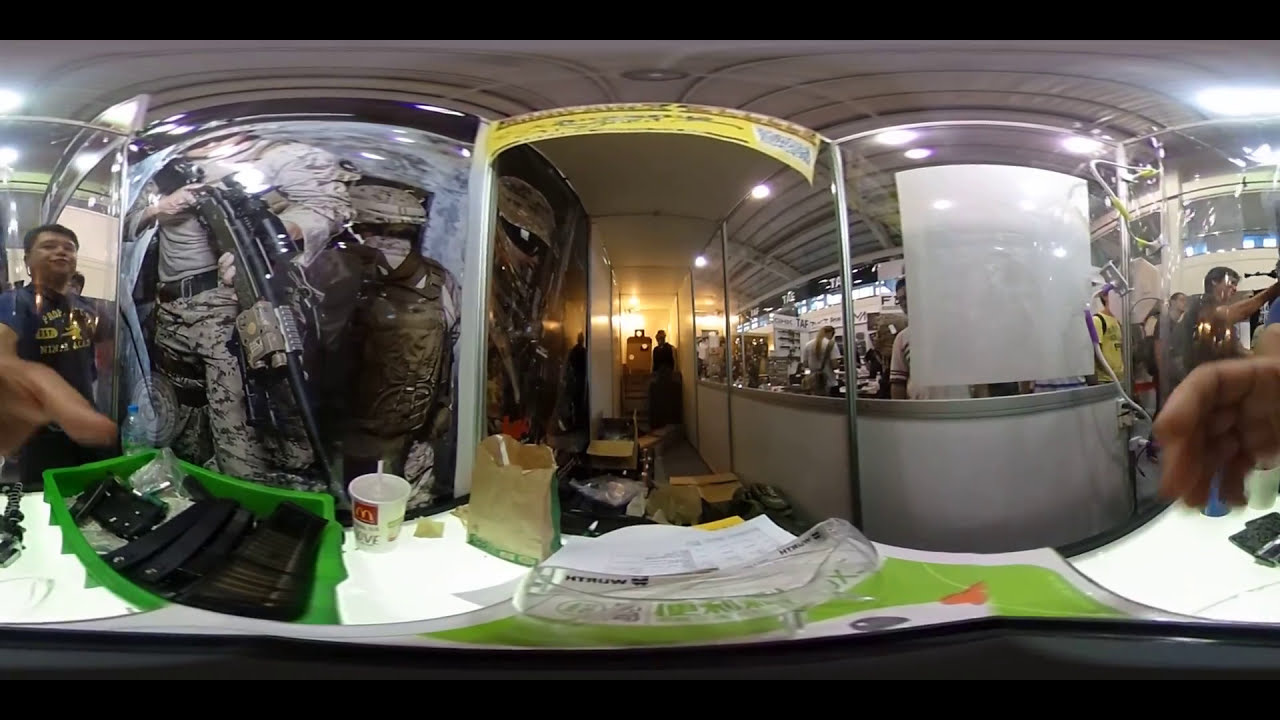The image captures a panoramic, 360-degree view of what appears to be a gun range or a military-themed store/museum. On the far left, a man in a blue t-shirt with red lettering is seen in motion, possibly holding the camera, his dark hair and hand visibly extended. Adjacent to him is a glass case containing a mannequin dressed in camouflage attire, holding a large sniper rifle, with a military knapsack nearby. Moving to the center, there is a long hallway with white, rainbow-shaped striped ceilings and a yellow banner overhead, stretching into the distance. In the foreground stands a green bin filled with black ammo and a table cluttered with various items including papers, a McDonald's drink, and a paper bag. On the right side of the image, a man is attempting to lift something from the table, surrounded by what seems to be bullets and gun parts. Further back, another man is seen standing next to a dummy, potentially engaged in shooting practice. A glass panel on the right encloses several people and displays numerous firearms, adding to the military ambiance of the scene.